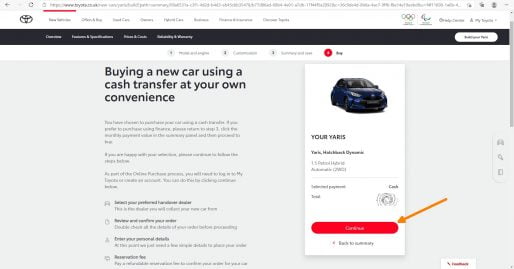A detailed screenshot of a web page, likely for a car brand (possibly Toyota based on the logo on the left side of the header). The logo is grey, with unreadable text beneath it. To the right of the logo are several menu boxes, also unreadable due to blurriness. At the very top of the page, there's a search bar indicating this is a website screenshot. Below the search bar and aligned with the menu boxes, there are additional blurred buttons on the left. Below this line, there is a black text box with four options in white font, stretching from left to right. The rightmost option seems to be a button, though the text is not legible.

On the next line, centered options are present, and one has a red circle next to it, perhaps indicating an important link or button, possibly labeled 'buy' due to its short length. Below this is the main ad content, prominently displaying the text: "Buy the new car, use a cash transfer at your own convenience." This section includes three more paragraphs and several bullet points, all centrally aligned.

To the right of this text is an image of a car with the label "Your Yaris" and some accompanying information. There's a red button next to the car image, highlighted by an arrow, although the button's purpose is not specified. The car and its details are within a white text box on a grey background, which also contains blurred-out text that could potentially include an address or pricing details.